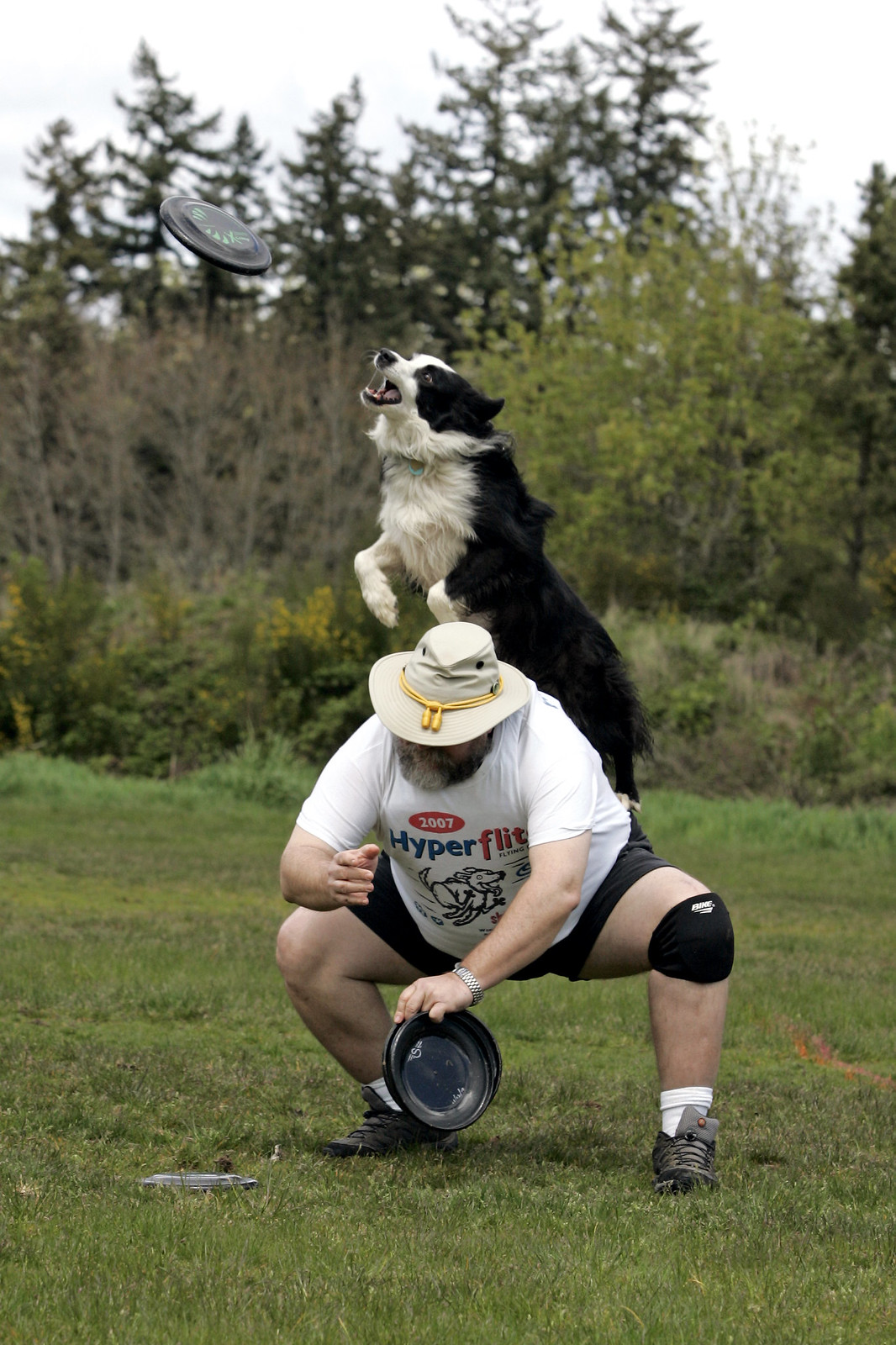In this vibrant, vertically oriented color photograph, we are outdoors on a somewhat cloudy day in a lush, grassy field framed by dense green trees and shrubs. The image centers around a playful interaction between a heavyset, older man and his energetic black-and-white long-haired dog. The man, sporting a beige floppy hat with a gold cord, dark shorts, white socks, brownish-green tennis shoes, and a white t-shirt with a logo featuring red and blue text, is crouched down on his feet and heels, with a black knee brace on his left knee. He holds one black Frisbee in his hand while another Frisbee can be seen flying through the air in the dog's direction.

The poised dog, mid-leap with its back legs on the man’s back, has white fur on its belly, paws, chest, and part of its face, with black fur adorning its back, ears, and the sides of its face. The dog’s mouth is open, revealing its pink tongue and bottom teeth, its whiskers are visible around its snout as it aims for the airborne Frisbee. The dynamic composition captures the exhilarating moment just before the dog attempts to catch the Frisbee, showcasing the teamwork and playful bond between the man and his canine companion.